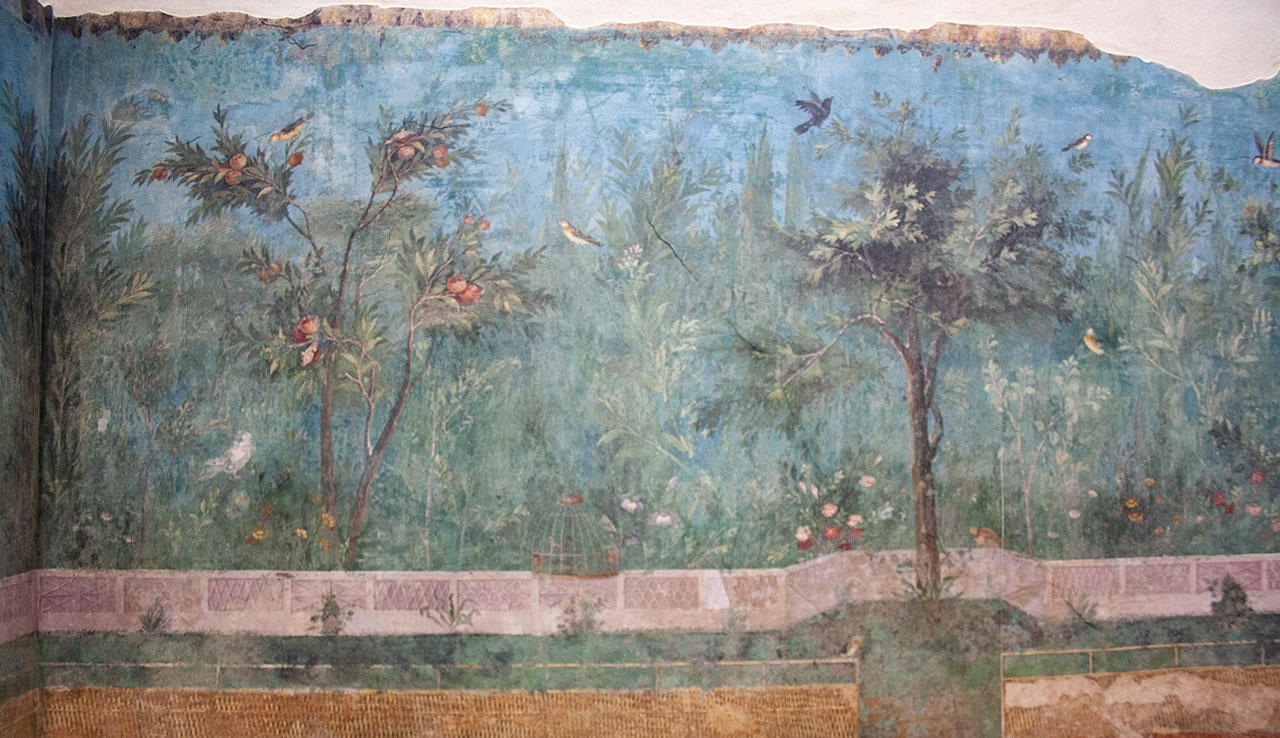This image showcases an intricate and large wall painting depicting a mesmerizing nature scene. Dominated by a realistic and artistic style, the mural features a variety of trees, including a notable large maple tree and a willow tree. The trees are lush with green foliage and vibrant fruit—some appear to be peaches with pinkish-orange hues while others look like apples. Birds are a prominent feature; some are gracefully flying while others perch within the trees. The foreground of the painting displays colorful flowers adding to the garden-like ambiance. Below this lush scenery, there's a detailed section with a terracotta-colored stone border that includes intricate grating. Beneath this, a wicker fence-like structure runs across the bottom. A golden and red birdcage also adds an interesting focal point within the scene. The top part of the wall painting shows a blue sky background, which appears slightly imperfect and peeling in areas, adding character to the artwork. Additionally, there are subtle shadows and faded-out leaves in pale grayish-green and yellow tones in the background, contributing depth to this long and visually rich mural.